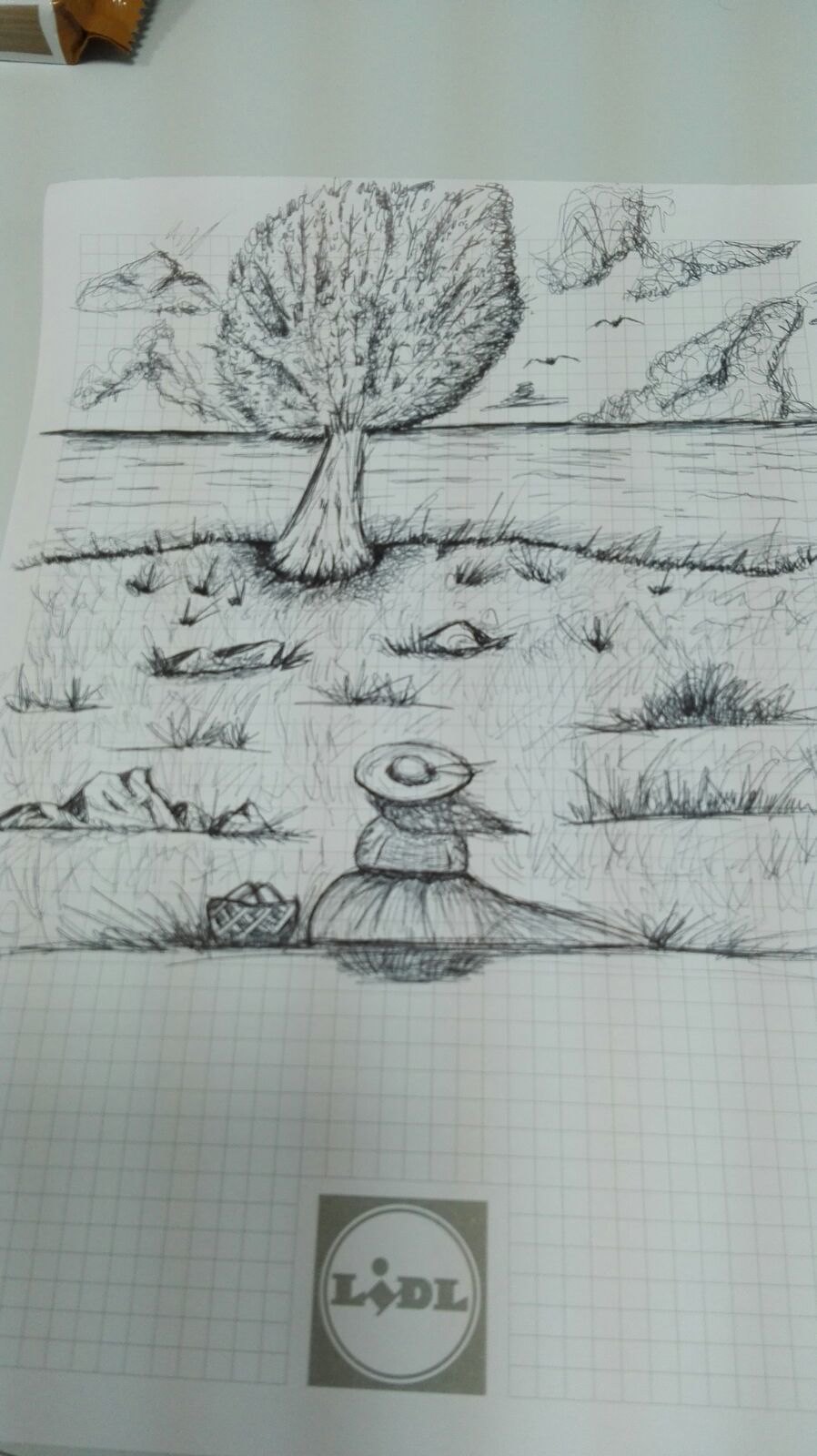This charming, almost childlike drawing is sketched on squared paper, giving it a quaint, old-fashioned feel. Central to the composition, albeit slightly askew at the bottom, is a square sign displaying the Lidl logo. In the near foreground sits a small girl, viewed from behind, who wears a straw hat and holds a basket. She is perched on a gently sloping grassy bank, gazing serenely towards a meandering river. The landscape around her features undulating terrain with tufts of grass, various plants, and occasional rocks. To her left, a large tree with a rounded canopy dominates the scene, while the background reveals a picturesque mix of rocks, trees, and bushes lining the opposite riverbank. The overall style of the drawing is naive, evoking a sense of innocence and simplicity.